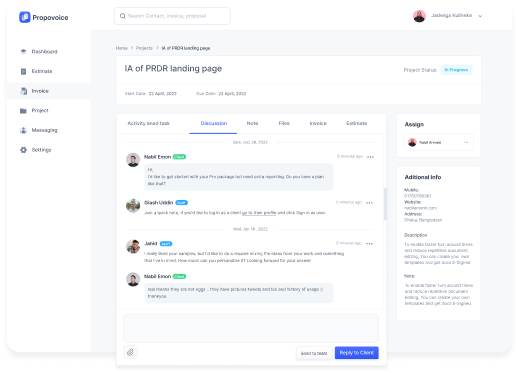The image depicts a nearly square-shaped webpage layout featuring a user interface for a website or web application. The layout consists of a vertical sidebar on the left and a horizontal header at the top. 

The left sidebar contains the website's main navigation menu and begins with a blue box at the top left corner, which has a small, indistinguishable white emblem inside. The text "Purple Wolfs" is visible beneath this emblem. Under the website name, a list of menu options is vertically organized, including "Dashboard," "Invoice," "Project," "Managing," "Settings," and another slightly unreadable option that appears to be "Essentials," each accompanied by small icons.

The top horizontal banner includes a search box labeled "Search here," a circular user profile picture, and some adjacent text which is unclear in the given image. 

The main content area of the webpage has a partially visible heading that reads "IA of PRDR Landing Page," although the smaller print in this section is too tiny to decipher. 

Additionally, another horizontal menu with six menu items spans across the top of the main content area. The menu item "Discussion" is selected, highlighted in blue, and underlined, indicating it is the current active section.